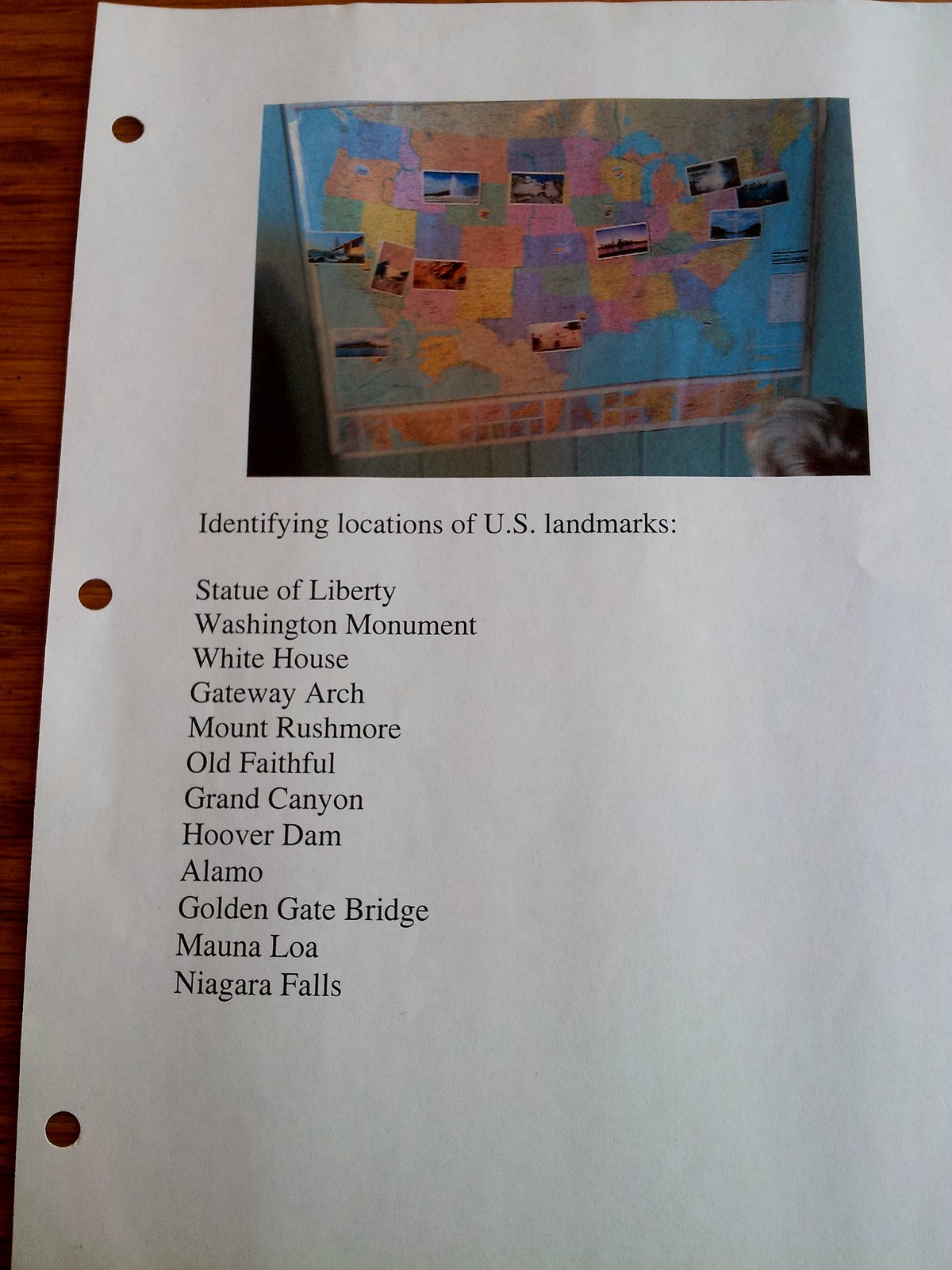This photograph captures a white piece of paper that has been hole-punched on the side to fit into a binder. Centered at the top of the page is a map of the United States, adorned with various images of significant landmarks located across different regions. Immediately beneath the map, in bold black text, the heading reads, "Identifying Locations of U.S. Landmarks." Following this heading, there is a neatly organized list, also in black text, that enumerates the landmarks as follows: Statue of Liberty, Washington Monument, White House, Gateway Arch, Mount Rushmore, Old Faithful, Grand Canyon, Hoover Dam, Alamo, Golden Gate Bridge, Mauna Loa, and Niagara Falls.